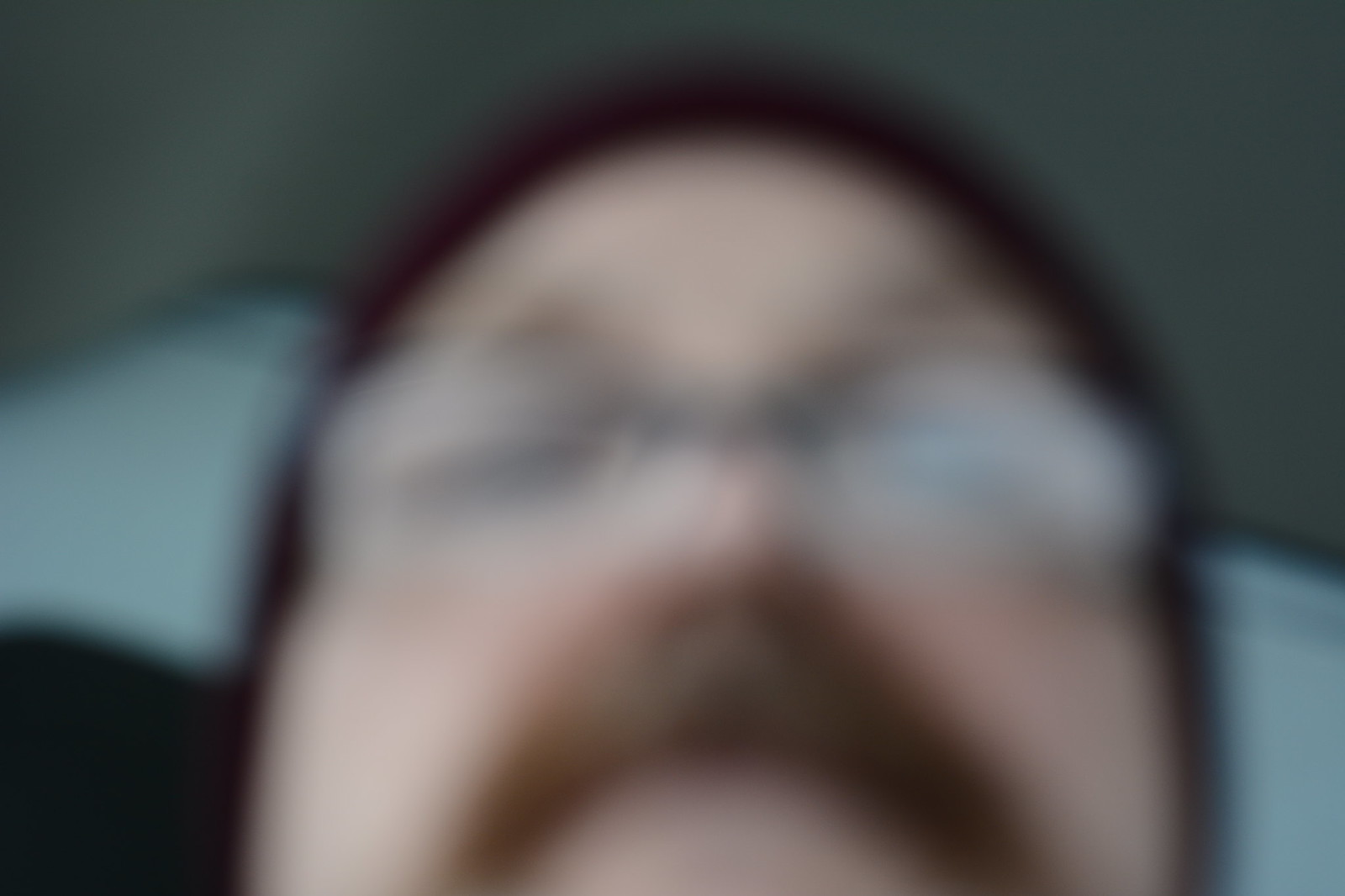The photo is extremely blurry and out of focus, but it clearly depicts a close-up of a man's face. The man, likely a fair-complexioned Caucasian in his 30s or 40s, has short hair and is wearing glasses. He sports a large, thick mustache that stretches from his nose to the edges of his mouth, resembling a walrus mustache with a reddish-brown hue. The man appears to be heavyset, with a round face and rosy cheeks and nose. He's possibly wearing a hat—either a reddish-brown cap or a black beanie. The photo, potentially a selfie, seems to be taken from slightly below the man's face, capturing an upward angle. The background is a mix of colors with a dark green section behind him, a white section below, and a dark blue or black area in the lower left-hand corner.